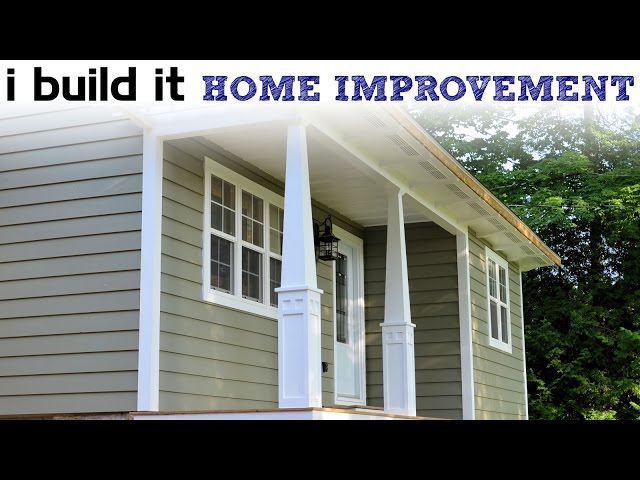The image showcases a picturesque, traditional house nestled in a lush, wooded area. The house, with its light olive-green and white exterior, features grey vinyl siding complemented by white trim. At the front, a small porch is supported by two white, tapering columns that add to the inviting appearance. The porch also includes a central white door with a glass window and flanked by two matching white-framed windows. The porch ceiling is white, seamlessly blending with the trim. Towering green trees gracefully envelop the house, enhancing its serene forest setting. Above the house, the image carries the text "iBuildit Home Improvement," with "iBuildit" in black font and "Home Improvement" in a navy blue, stone-textured font. This layout suggests that the image is likely used as a thumbnail for a video or a banner for a home improvement contractor advertisement. Black borders at the top and bottom frame the image, adding a well-defined look.